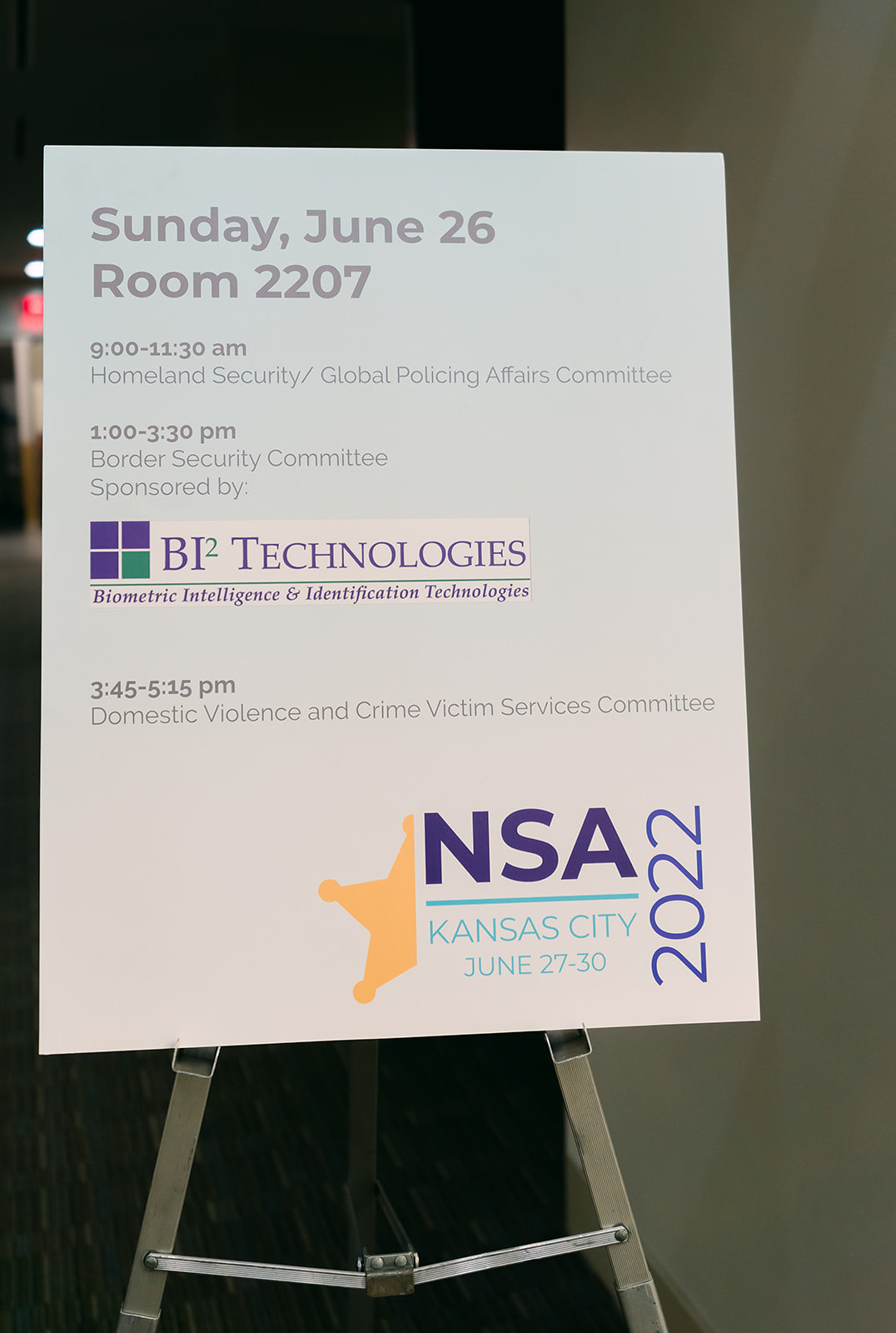The image depicts a standing sign attached to a metal easel or tripod, situated in what appears to be a hotel conference area. The sign provides detailed information about scheduled events on Sunday, June 26, taking place in Room 2207. At the top of the sign, in light gray text, it lists the date and room number. Below, from 9:00 to 11:30 AM, it mentions the "Homeland Security Global Policing Affairs Committee," followed by the "Border Security Committee" from 1:00 to 3:30 PM, which is sponsored by BI2 Technologies (Biometric Intelligence and Identification Technologies). Further down, from 3:45 to 5:15 PM, it references the "Domestic Violence and Crime Victim Services Committee." In the lower right corner of the sign, there is a partially visible sheriff-like star emblem next to the text "NSA Kansas City, June 27-30, 2022." The background reveals a white wall to the right, a carpeted floor below, and an exit sign, suggesting a hotel setting. The ceiling, shown at the top left of the image, is a dark gray.